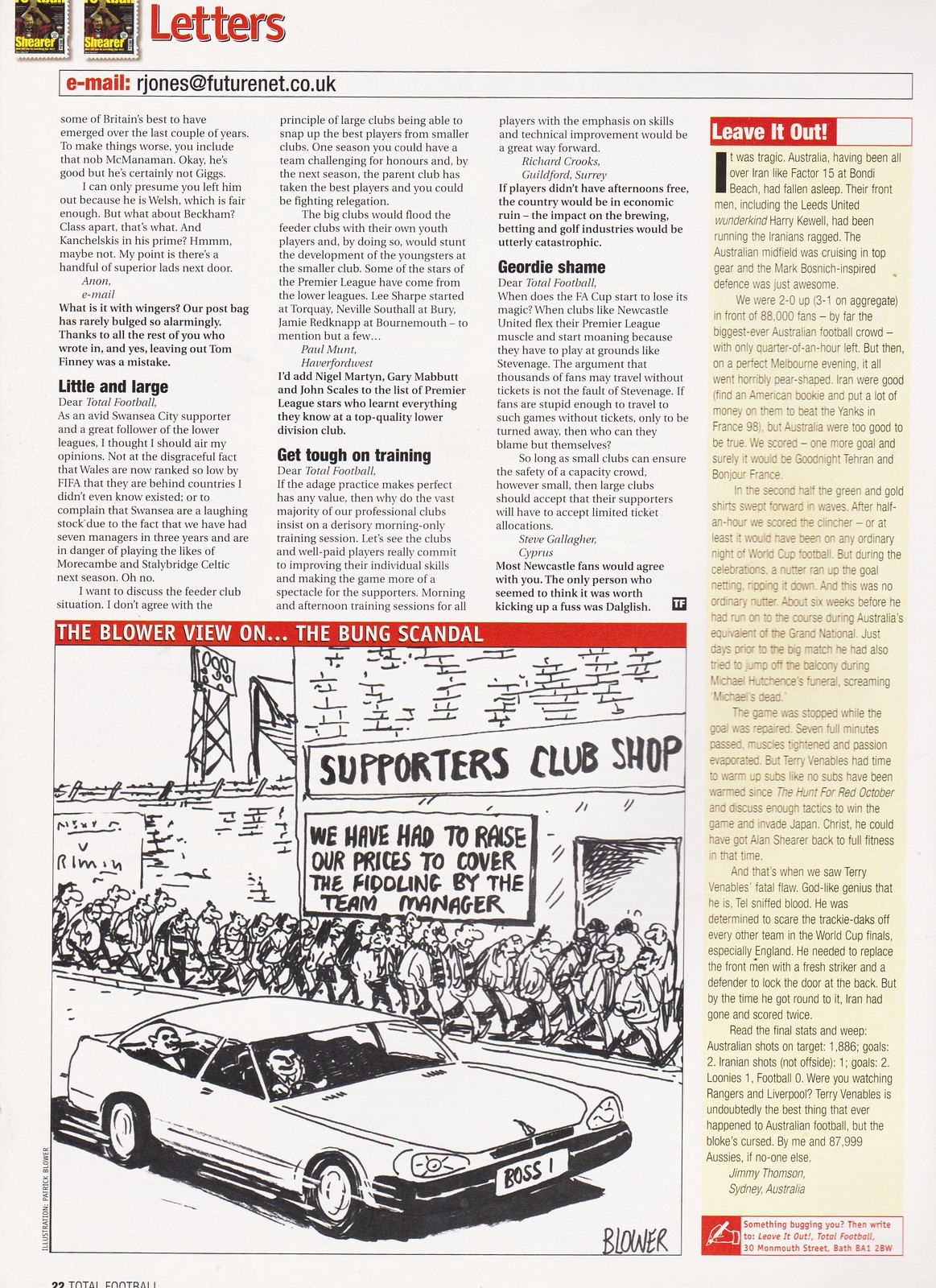A detailed page from a magazine titled "Letters" features multiple reader submissions, but its standout element is a prominent cartoon in the lower left-hand corner. This cartoon, taking up about half of the page, is set against a backdrop of a brick building labeled "Supporters Club Shop." A sign humorously declares, "We have had to raise our prices to cover the fiddling by the team manager." Above the cartoon, in a red strip with white lettering, reads, "The Blower View on the Bung Scandal."

In the cartoon, a long line of people, looking sorrowful and disheartened, queues to enter the shop. Parallel to the line, a limousine with a license plate that reads "BOSS 1" is driven by a chauffeur, with a man in the backseat enjoying a cigar. The artist, "Blower," has signed the illustration in the lower right-hand corner. The page also includes a small vertical box on the right side with the heading "Leave it out," discussing an unrelated yet captivating anecdote about Australian football. The page number, either 22 or 23, and the magazine title "Total Football" are indicated at the bottom.